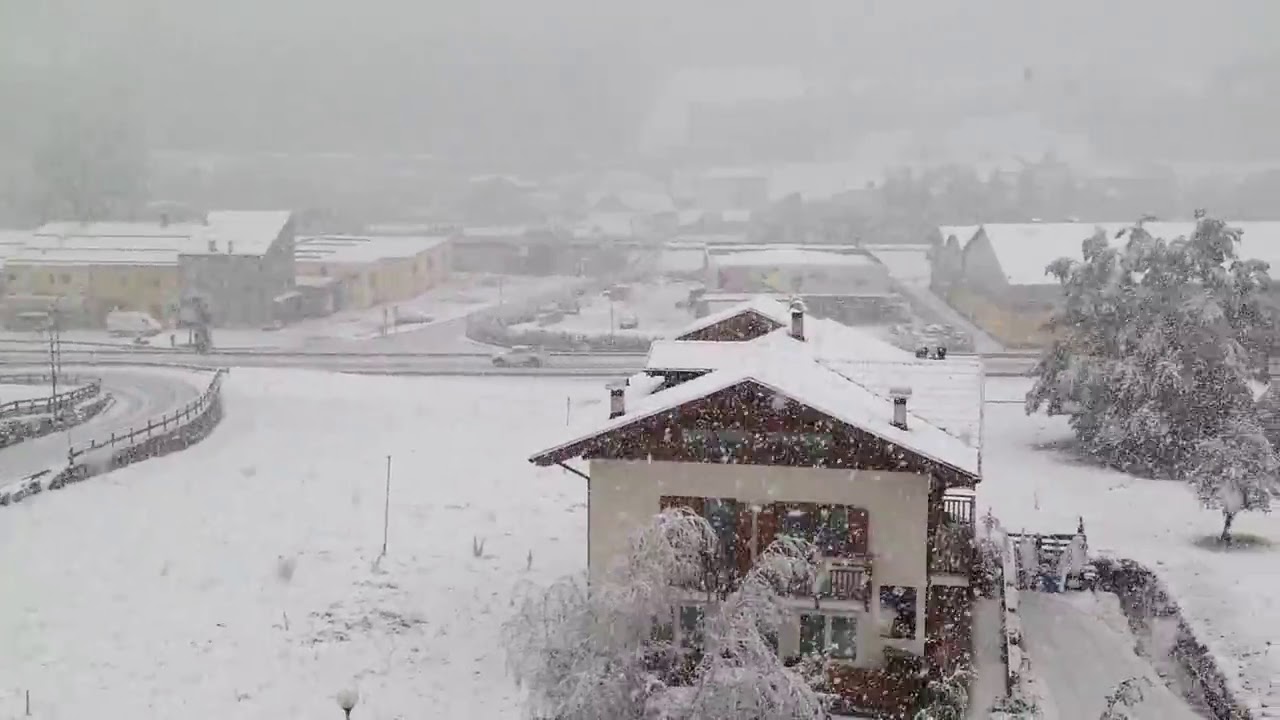This image captures an outdoor, elevated view of a small town enveloped in a heavy snowstorm. Dominating the foreground near the center, slightly to the right, is a light brown, two-story house with a snow-laden, slanted roof and three chimneys visible. The house sits within a large snow-covered yard and is bordered on the right by a sizeable snow-clad evergreen tree. A snow-blanketed driveway runs to the right of the house, leading to a road in the background where a white truck is distinctly visible, moving leftward through the snow. 

Further in the distance, other buildings, roads, and scattered cars are faintly discernible through the dense snowfall, which continues to obscure parts of the image. The top of the frame is dominated by a thick, smoky gray sky, enhancing the wintry atmosphere and making it difficult to see the city's outlines. On the left, a curved road edged by a snow-laden fence can be seen, also blanketed in white. The right side of the image features an enclosed backyard and more snow-covered trees, whose branches bear traces of frost. Overall, the scene is a picturesque, tranquil depiction of town life amidst a snowstorm, presenting a serene yet stark wintery landscape.